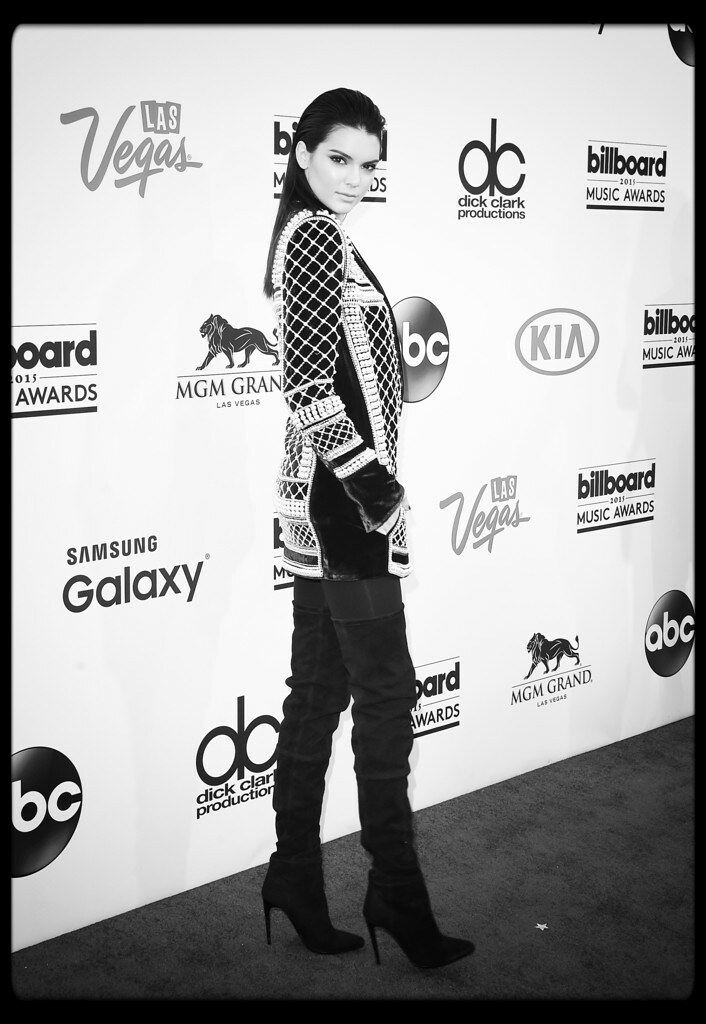In this black-and-white photo, an elegant actress is posing at the Billboard Music Awards 2021. She stands confidently before a backdrop adorned with logos such as Las Vegas, Dick Clark Productions, MGM Grand, ABC, Kia, and Samsung Galaxy. The actress is dressed in thigh-high black velvet boots with high heels, which accentuate her tall, lean frame. She pairs these with black leggings and a distinctive black jacket adorned with a white diamond lattice pattern that extends to the arms, front, and back. Her long, straight dark hair cascades down, framing her face. She gazes directly into the camera with a serious expression, while the star-studded wall behind her underscores the prestigious event. A small star emblem can be seen on the ground near her feet, adding a subtle touch of glamor to the scene.